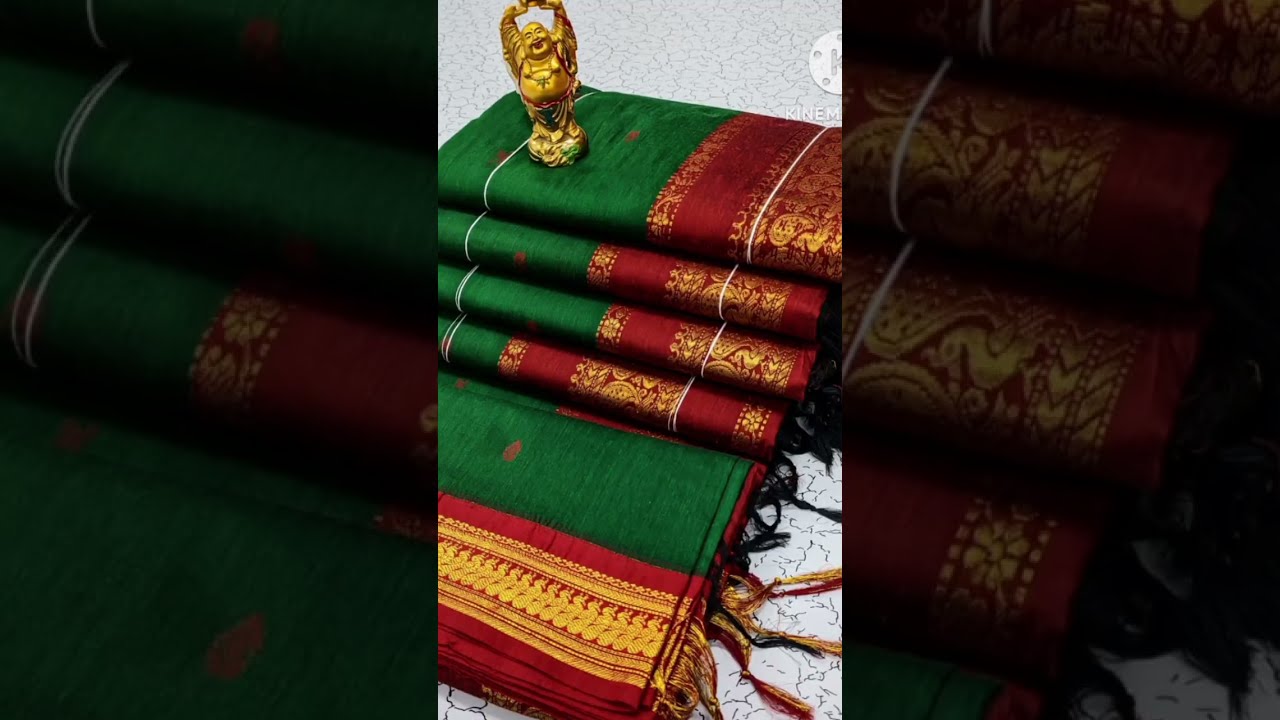In the center of the high-definition triptych image lies a detailed photograph featuring a beautifully arranged pile of saris on an outdoor, uniquely white tiled floor. The saris, primarily green with striking red borders, are richly adorned with gold embroidery and delicate tassels. Arranged in two bundles, the larger one comprising five saris is stacked beneath a smaller pile of one or two saris. Cord loops secure the fabric bundles, enhancing their layered presentation. Atop this ornate heap, a golden statue of a smiling Buddha, with arms raised in a gesture of joy, serves as the focal point. The image's central panel is flanked by two blurred, enlarged close-ups of the saris—the left panel focusing on the shiny green fabric and the right on the red border—creating a harmonious blend that accentuates the intricate details and luxurious textures of the traditional fabric.